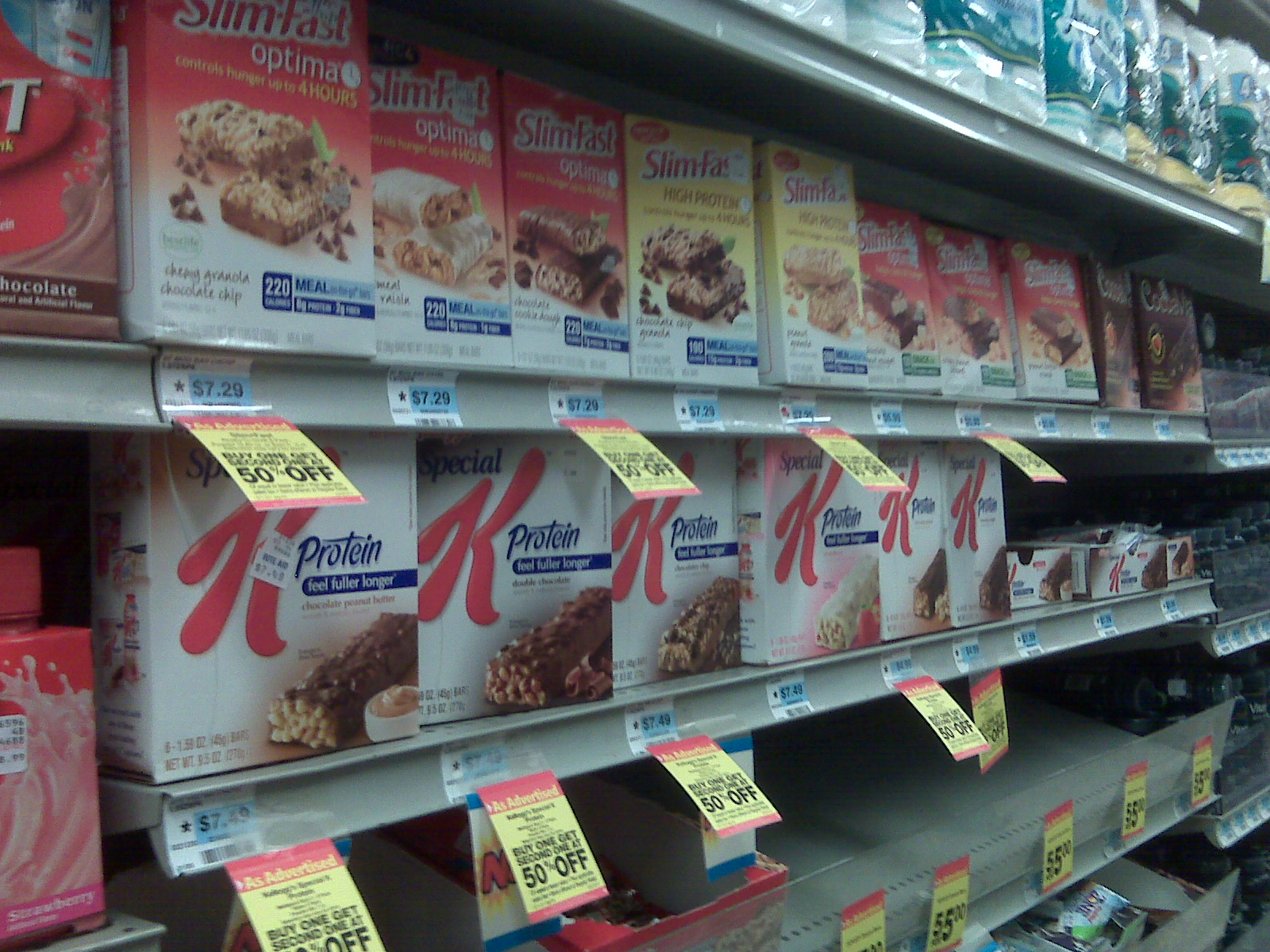This photograph captures a well-organized aisle in a supermarket, showcasing shelves packed from top to bottom with various products. The top shelf is stocked with rows of paper towels or toilet paper. Below it, the second shelf features an assortment of SlimFast Optima bars in different packaging colors, predominantly in red, with some yellow and brown. The third shelf is dedicated to a variety of Special K protein bars, including different flavors such as chocolate and those covered in white chocolate or yogurt. The fourth shelf from the top is notably empty, while the lowest visible shelf contains unidentifiable items. Sprinkled amongst the second and third shelves are numerous bright yellow and red tags proclaiming a promotion: "Buy one, get the second one at 50% off." The shelves themselves are a mixed hue of yellow, off-white, or tan, adding to the overall neat and inviting presentation of the products.